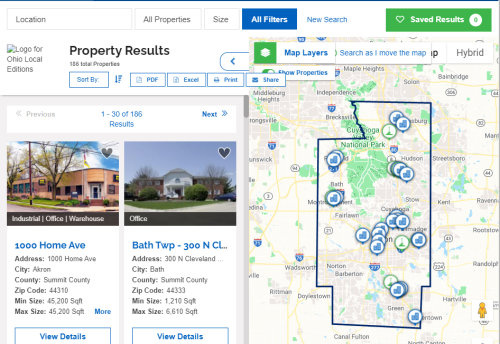This is an image of a property search interface focused on real estate listings in Summit County, Ohio, specifically in the areas of Akron and Bath. The screen displays the results from a search performed on the "Ohio Local Additions" platform. At the top of the interface, there is a search bar allowing users to input a specific location, with additional options for filtering properties by size and other criteria. Key filters include "All Properties," "Size," and an "All Filters" button, which is highlighted in blue. A "Saved Results" option is also visible, marked in green.

The main section of the screen reads "Property Results" and indicates that it is displaying items 1 to 30 of a total of 186 results. Each property listing provides detailed information, including the address, city, county, zip code, minimum size, and maximum size of the property. A "View Details" button is present at the bottom of each listing for more in-depth information. Currently, only two property listings are visible, but the interface appears designed for scrolling to access additional entries.

To the right of the listings, a map showcases the geographic locations of the properties within the specified search area. The map prominently includes landmarks such as Cuyahoga Valley National Park, various roads, waterways, and small lakes, providing a comprehensive view of the surrounding environment.